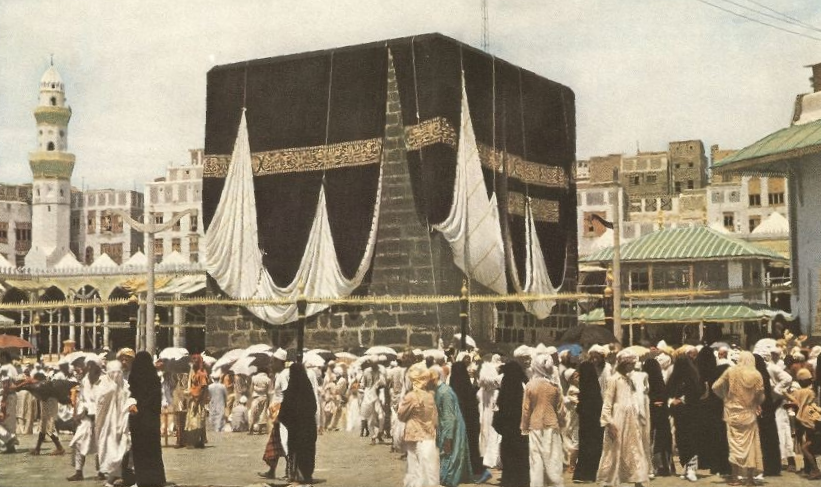The photograph depicts an older image of Mecca, prominently featuring the Kaaba, a sacred Islamic site situated at the center of the Majid al-Haram mosque. The image is muted in color, suggesting that it is dated. The Kaaba appears as a distinct black cube with golden lettering on its edges, draped in a black cloth, some parts of which are lifted or lowered, revealing a white inner side. Surrounding the Kaaba is a bustling scene of many people, indicating the traditional practice of walking around the Kaaba as part of their pilgrimage. 

The crowd includes men dressed predominantly in long white robes and a variety of headgear such as turbans, headbands, and even umbrellas. Among them are women fully covered in black burqas, some of whom are accompanied by men. The faces of the people are diverse in complexion, ranging from light brown to very dark brown. 

Encircling this central activity is a cityscape of Mecca, featuring Middle Eastern architectural designs. On the left side, a towering white spire of a mosque stands out, while to the right, the buildings vary in distance and elevation, some forming a diverse urban landscape, likely hinting at structures built on hills. The overall scene portrays a significant yet less crowded moment in the history of this sacred place, reflecting a time when fewer people could undertake the pilgrimage to Mecca.